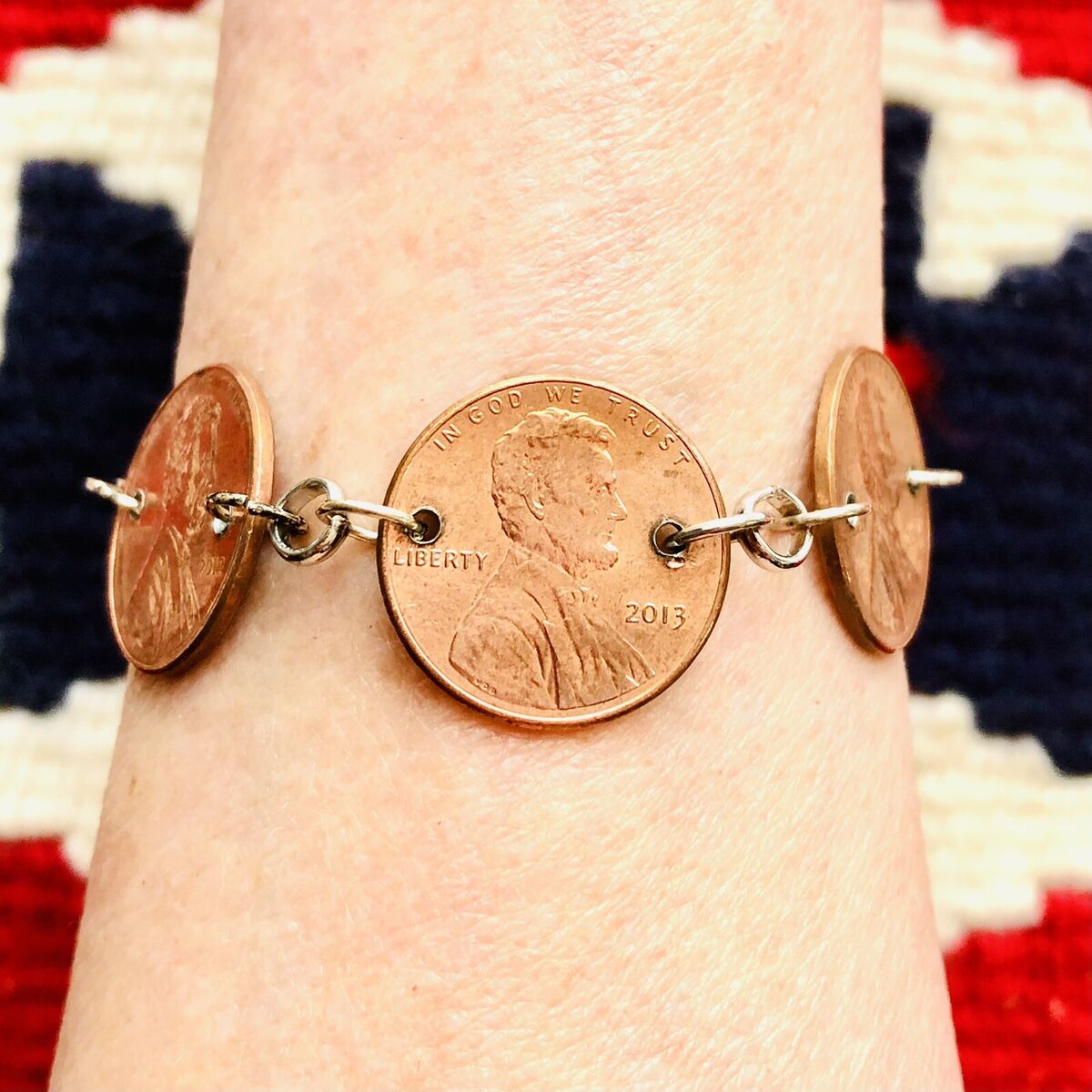The photograph showcases a close-up of a Caucasian person's wrist adorned with a unique, handcrafted bracelet composed of copper pennies. Each penny, including a prominently featured 2013 penny inscribed with "In God We Trust" and "Liberty," bears the iconic bust of Abraham Lincoln. Holes have been meticulously drilled on either side of Lincoln's face, through which metal loops are threaded. These loops are interlinked with small silver chains, creating a continuous bracelet. Visible on this side of the wrist are three pennies, suggesting there may be more completing the bracelet around the wrist. The background fabric displays a red, white, and blue pattern, hinting at the possibility of it being an American flag or similarly themed material. The overall scene reflects a blend of creativity and patriotism.